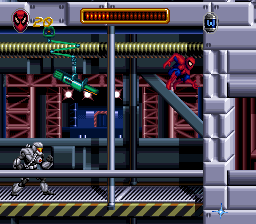The screenshot depicts a video game screen, showcasing a small, square image. At the center of the action, Spider-Man is featured, poised mid-jump on a diagonal metal pole. The background includes a series of red triangles and rectangles, whose function is unclear. On the left side, a character clad in silver armor appears to be running on what looks like a conveyor belt. In the top-left corner, Spider-Man's head icon is visible next to the yellow number "29" or "20." Across the middle-top of the screen, a bar outlined in yellow with red dashes is displayed. Spider-Man seems to be attempting to enter a structure made of silver-gray bricks.